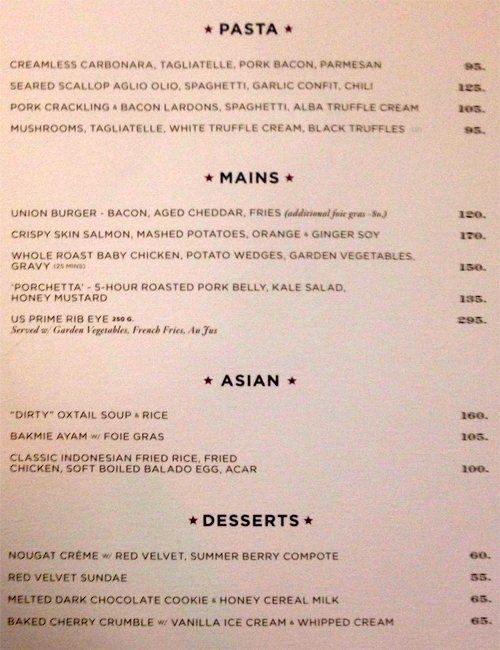This menu, printed on cream-colored paper with black lettering, is organized into several sections featuring a variety of dishes. At the top, under the "*Pasta*" section, you'll find four enticing dishes: Creamless Carbonara with pork bacon and parmesan priced at 95, Seared Scallop Aglio Olio Spaghetti with garlic confit and chili priced at 125, Pork Crackling Bacon Lardon Spaghetti with Alba truffle cream for 105, and Mushrooms Tagliatelle with white truffle cream and black truffles at 95.

Following the pasta section, the "*Mains*" section offers a tempting selection that includes the Union Burger with bacon, aged cheddar fries, and an option for foie gras at 120, Crispy Skinned Salmon with mashed potatoes, orange, ginger, soy for 170, Whole Roast Baby Chicken with potato wedges and garden vegetables (accompanied by gravy) for 150, Porchetta—five-hour roasted pork belly with kale salad and honey mustard—at 135, and the U.S. Prime Rib served with garden vegetables, french fries, and au jus at 295.

The "*Asian*" section features three distinctive dishes: Dirty Oxtail Soup served with rice for 160, Bakmi Ahum with foie gras for 105, and Classic Indonesian Fried Rice with fried chicken, soft-boiled Bolado egg, and acar at 100.

Lastly, the "*Desserts*" section presents a delightful end to your meal with Nougat Cream topped with red velvet and summer berry compote at 60, Red Velvet Sundae for 55, Melted Dark Chocolate Cookie with honey cereal milk at 65, and Baked Cherry Crumble with vanilla ice cream and whipped cream also priced at 65. This detailed menu caters to a wide range of culinary preferences, ensuring a satisfying dining experience for all.